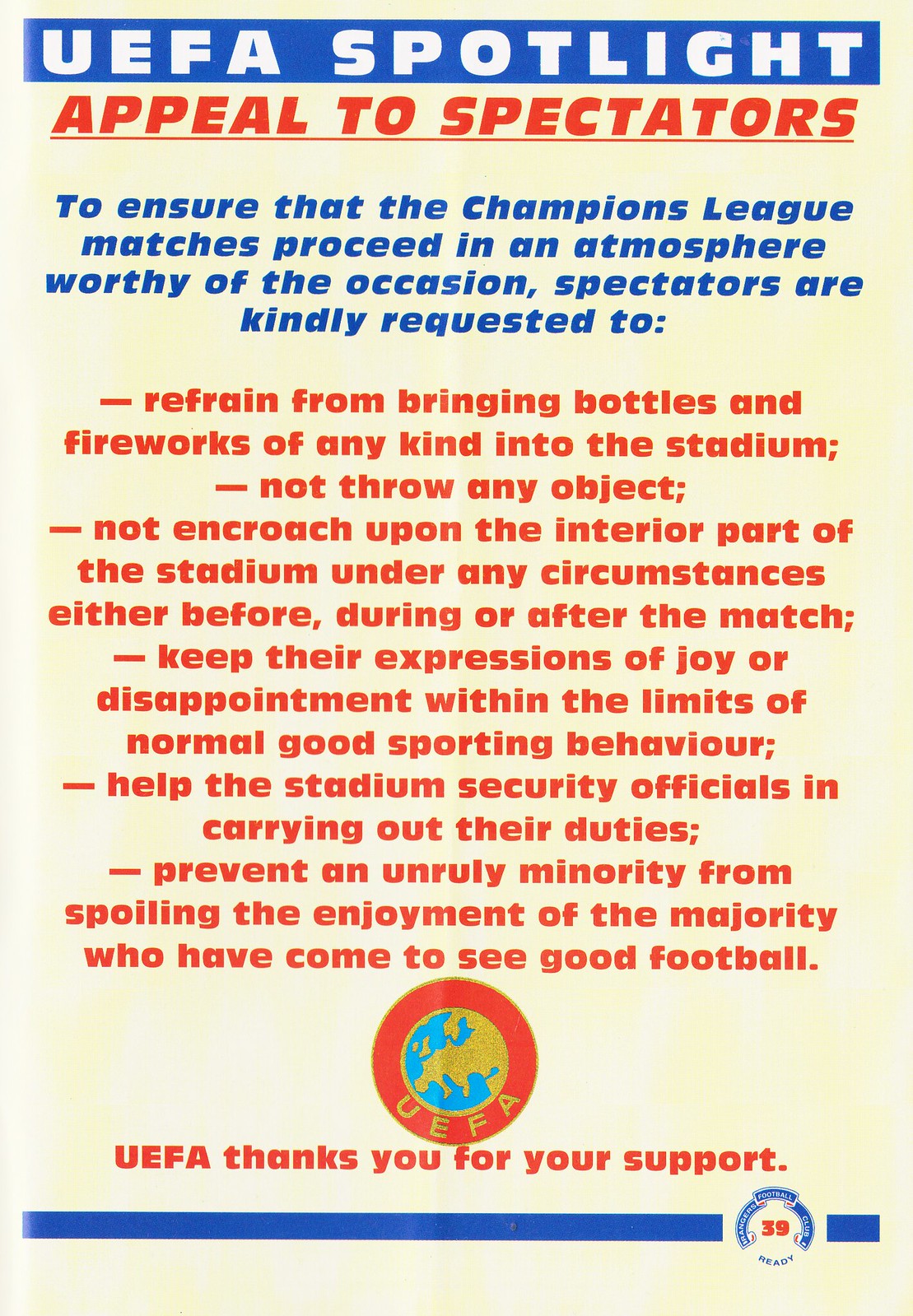This colorful and detailed poster, prominently displayed at soccer events across the European Union, is designed to convey important information to spectators. The top of the poster features the title "UEFA Spotlight" in bold white text set against a blue background. Below that, in vibrant orange letters, is the heading "Appeal to Spectators." The text beneath outlines the regulations for ensuring that the Champions League matches proceed in an appropriate and respectful atmosphere.

Spectators are kindly requested to refrain from bringing bottles and fireworks of any kind into the stadium, not to throw any objects, and not to encroach upon the interior part of the stadium under any circumstances, whether before, during, or after the match. Patrons are also urged to maintain their expressions of joy or disappointment within the bounds of normal good sporting behavior, to help stadium security officials in carrying out their duties, and to prevent an unruly minority from spoiling the enjoyment of the majority who have come to see good football.

A rust-colored round emblem featuring a depiction of a map symbolizing UEFA, including regions like Great Britain, is placed beneath the text. At the bottom of the poster, in orange letters, is the message, "UEFA thanks you for your support," underscored by a blue line. The background of the poster is generally yellowish, with text in white, red, and blue fonts, creating a visually striking and informative appeal to all match attendees.